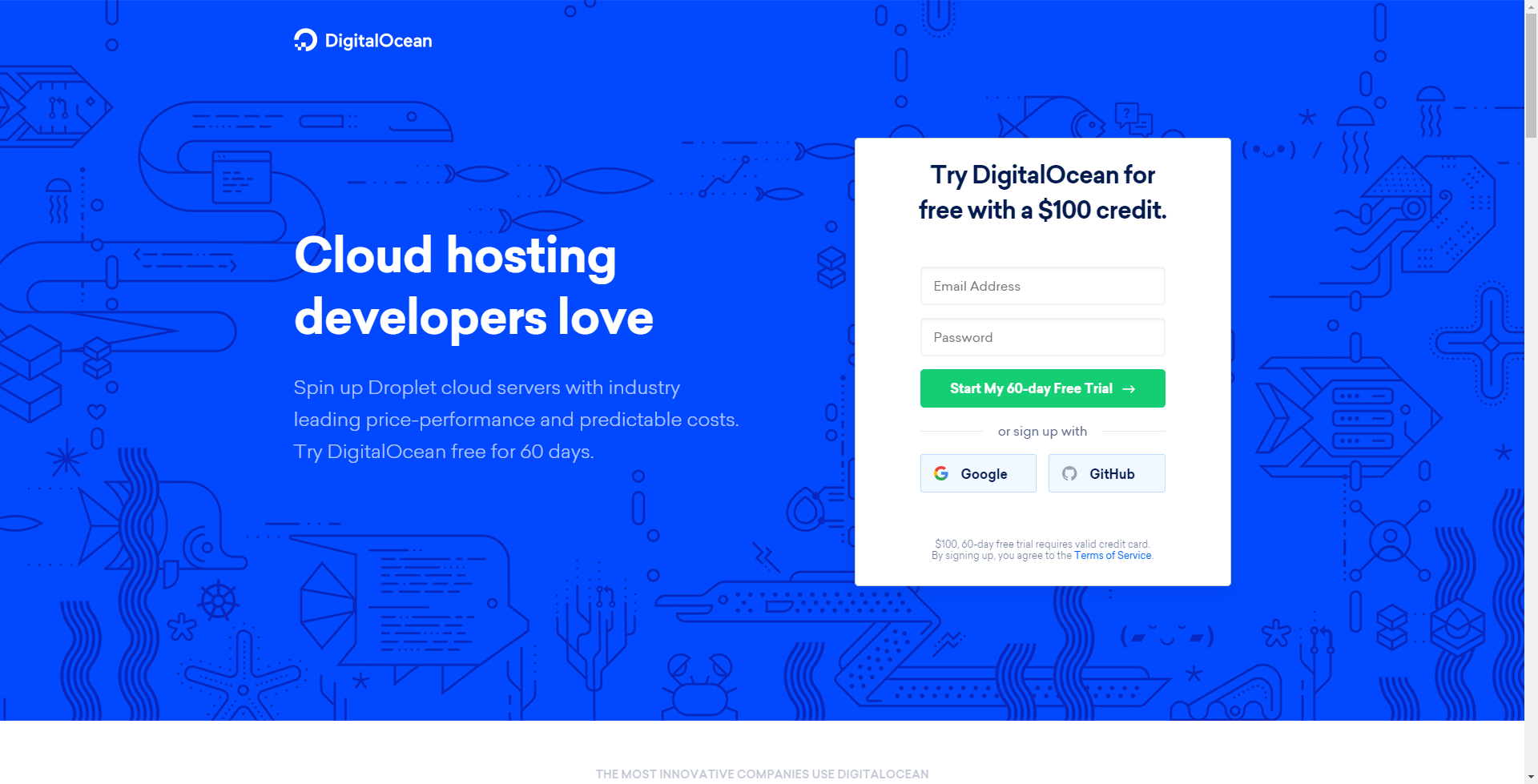A screenshot captured from a desktop or laptop showcases a website with a distinctive underwater theme, featuring a dark yet vibrant blue background adorned with illustrations of fish and other sea creatures, reminiscent of Etch-A-Sketch drawings. At the top of the screenshot is the DigitalOcean logo, composed of white text and a circular emblem. Below, larger white text reads: "Cloud Hosting Developers Love." Accompanying this is a promotional message: "Sign up, spin up, and deploy cloud servers with industry-leading price performance and predictable costs. Try DigitalOcean free for 60 days." Adjacent to the message is a white input box for entering an email address and password to start a 60-day free trial, which includes a $100 credit. Alternatively, users can sign up using their Google or GitHub accounts by clicking the provided buttons.